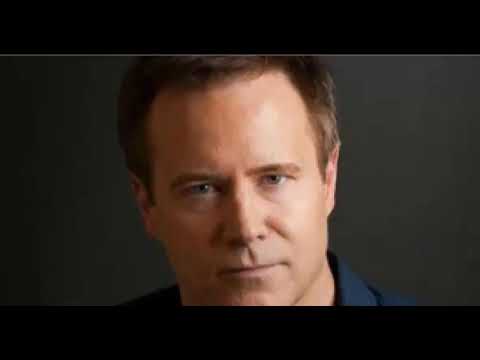The image is a square close-up shot of a middle-aged white man’s face, positioned against a charcoal-colored background with a gradient effect that is darker on the left and lighter on the right, particularly in the upper right-hand corner. The background is bordered by two thick black strips at the top and bottom edges. The man, who is in his 40s or 50s, has short brown hair with some faded gray on the sides, brown eyebrows, and blue eyes that might appear slightly blurry. His expression is neutral, and his head is centered in the frame, with his clean-shaven face taking up most of the image. He is wearing a navy blue collared shirt, and only the top of his shoulders and part of his chin are visible, the latter being cut off by the edge of the image. There is no text or additional elements in the image—just the man’s face, calmly staring directly at the viewer.